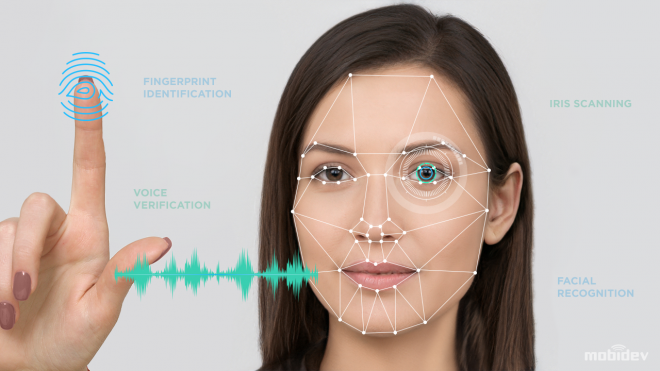The image features a CGI woman with long brown hair, an olive skin tone, and distinct heterochromatic eyes—one brown and one blue. Her face is covered with white diagram points illustrating facial recognition technology. She holds her hand up, pointing at a digital interface with her finger, which is encircled by a fingerprint identification marker. The image also displays various security verification methods: "fingerprint identification," "voice verification," "facial recognition," and "iris scanning" with a green circle over one of her eyes. The background is gray, and the woman is adorned with brownish-wine nail polish. The text "Mbiv" suggests the company's name, highlighting their suite of biometric security features.